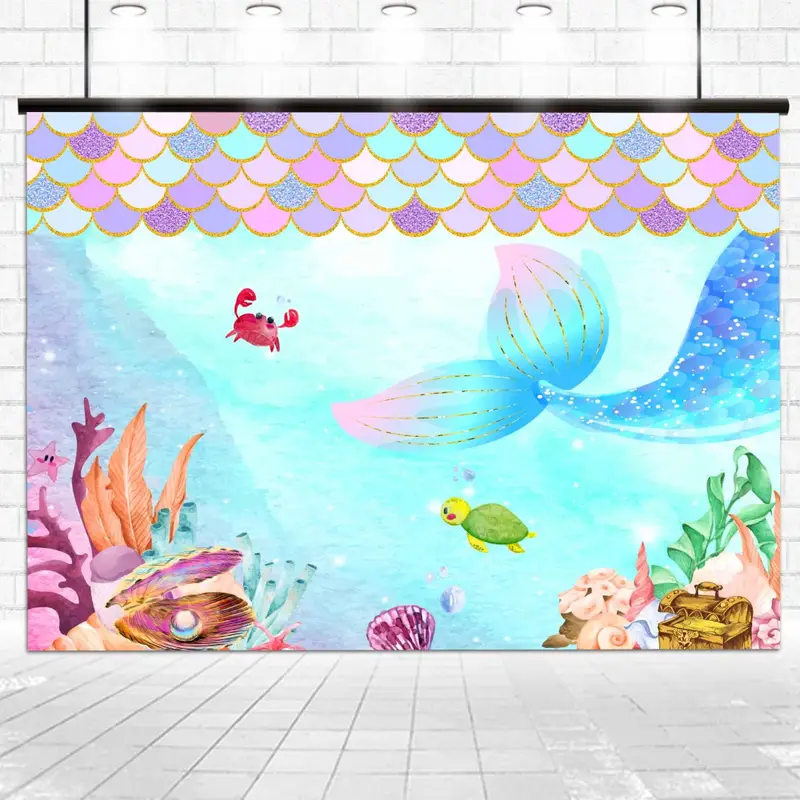The image depicts an underwater scene that appears to be either computer-generated or painted, hanging from two black holders against a gray painted brick wall background. It measures approximately six inches by six inches and is framed by a black horizontal bar at the top, resembling a projector screen. The top quarter of the image is adorned with semi-circle scales in shades of pink, blue, and purple, some of which are accented with glitter and outlined with gold glitter.

In the middle of the image, a whimsical underwater tableau unfolds: On the right, a blue and purple mermaid tail with pink tips elegantly dips into the blue water. A yellow and green turtle swims nearby, adding life to the scene. To the left, a red crab crawls amidst a vibrant coral reef. At the bottom, a treasure chest is nestled among seashells, with an open oyster revealing a shining pearl. The stylized art, rich in detail and vibrant colors, suggests an enchanting aquatic environment, making it a delightful decoration for a child's room or bathroom. Surrounding the mural, the backdrop features wet-looking gray stone tiles on the floor and circular fixtures resembling lights or showers at the top.